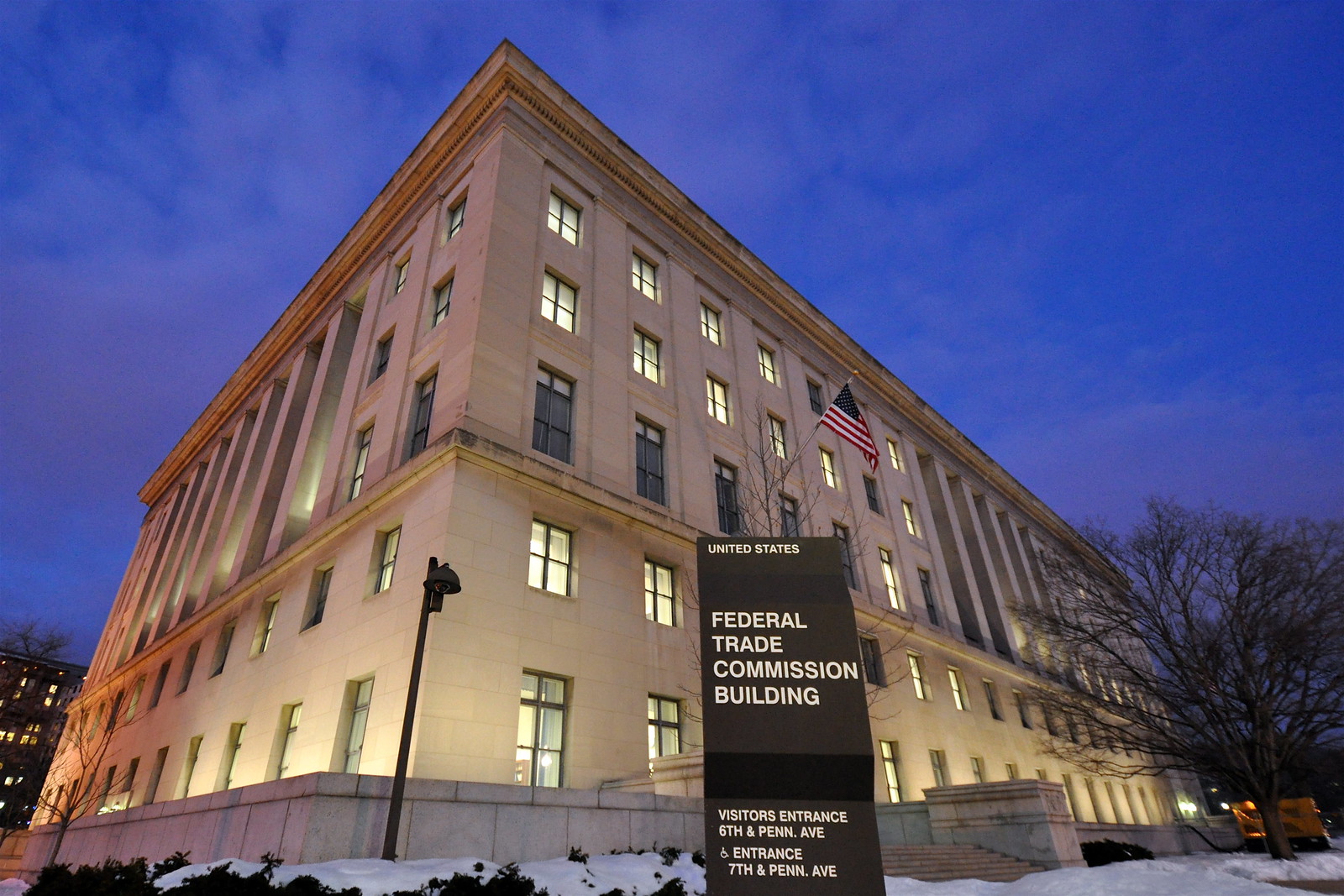This photograph captures the United States Federal Trade Commission (FTC) building during the serene, twilight hours just after dusk. The towering, beige stone structure is composed of five stories and features numerous rectangular windows, many of which glow with warm, yellow light from within. The sky above is a rich blend of violet and dark blue, with dark purple clouds hinting at the recent sunset.

In the foreground, a large, brown and black monolithic sign stands out, reading "United States Federal Trade Commission Building," along with directions for visitor and handicap entrances located on 6th and 7th Penn Avenue respectively. Snow blankets the ground, lending a quiet, wintry atmosphere to the scene. To the left side of the building’s entrance, a large, dormant brown tree stands stark against the stone facade.

An American flag is prominently displayed above the building’s door, adding a touch of patriotic resonance. Distant buildings are faintly visible in the background, softened by the diminishing light. Overall, the image conveys both the imposing presence and the elegance of the FTC building, accentuated by the snow and the fading twilight.